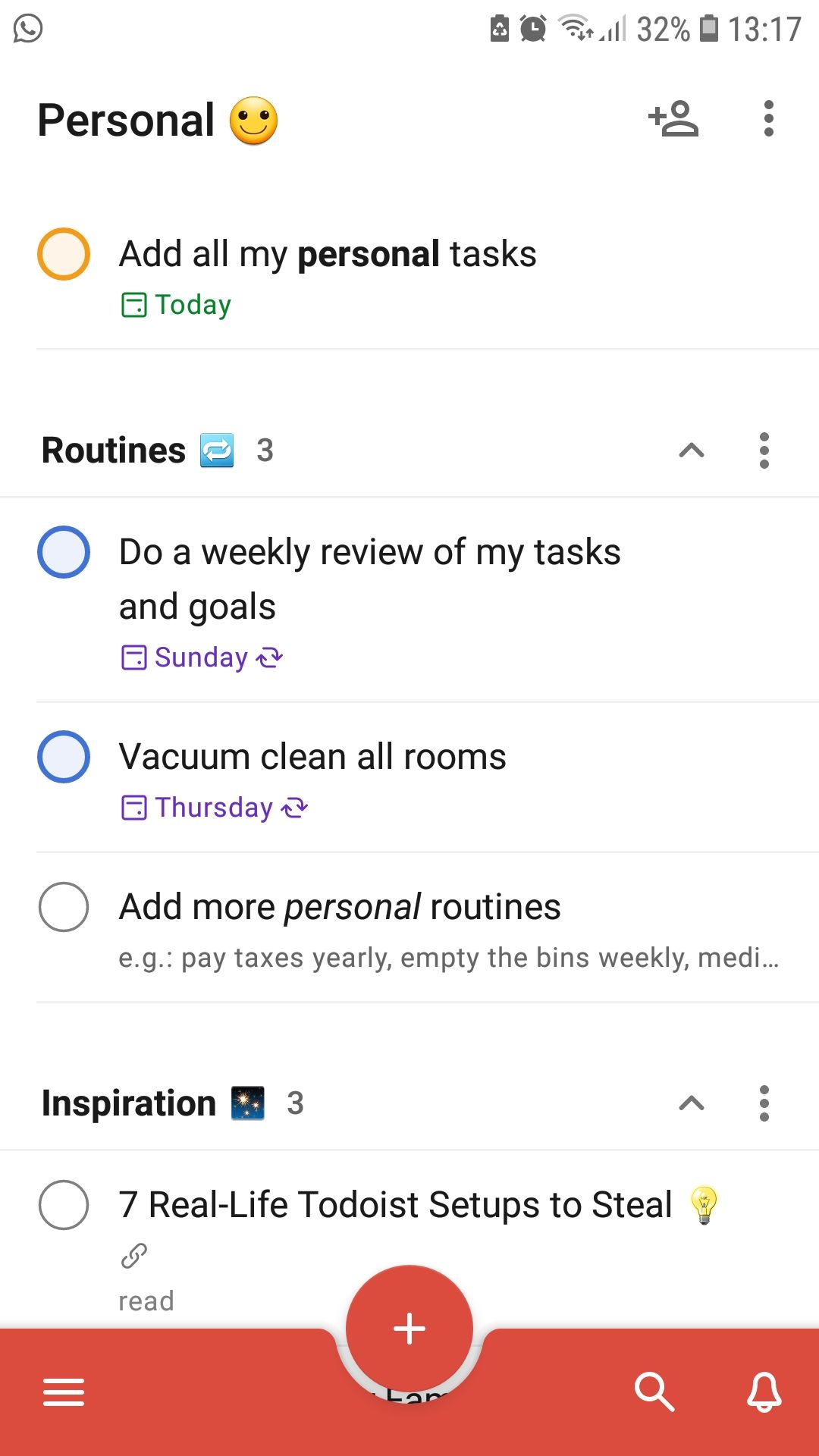**Screenshot of Personal Blackphone App Interface**

This screenshot captures the interface of the Personal Blackphone app, showcasing its task management features. 

At the very top right corner of the screen, standard cell phone status icons are visible, indicating signal strength, Wi-Fi connectivity, battery status, and other typical indicators. Directly below, the title "Personal Blackphone" is prominently displayed with a smiley face emoticon to its right, adding a touch of personalization.

The next section reads "Add All My Personal Tasks" followed by a header labeled "Today." There is a circular checkbox next to "Today," which has not been selected.

Following this is a section named "Routines," accompanied by a numeral "3," indicating the number of routine tasks listed within this category. 

The first routine under this category is "Do a Weekly Review of My Tasks and Goals," scheduled for "Sunday." A circular checkbox is present next to this task, but it remains unselected.

The subsequent task is "Vacuum Clean All Rooms," which is scheduled for "Thursday." Like the previous tasks, this one also has a circular checkbox next to it, which remains unselected.

Below these tasks, there is a prompt labeled "Add More Personal Routines," suggesting users can add additional tasks to their routine.

Finally, the last section is titled "Inspiration," hinting at another category or feature within the app likely dedicated to motivational content or quotes.